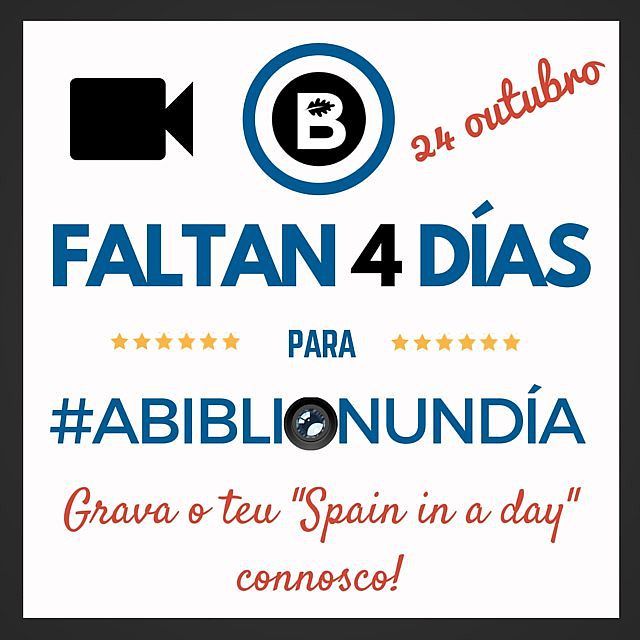This is a poster or banner advertisement, prominently featuring a white background with a black border. In the top left corner, there's a hand-drawn outline of a video camera facing right. Centered at the top is a circular emblem made up of three concentric circles: a blue outer circle, a white middle circle, and a black inner circle with a white "B" prominently displayed, featuring a leaf in the top hole of the letter. Next to this, in a red cursive script angled slightly upward, is 'OUTUBRO'.

Below this, in blue capital letters, it reads 'FALTAN 4 DÍAS', with the '4' in black and 'DÍAS' in blue. Underneath that, there is a row of six small yellow stars, the word 'PARA' in small blue letters, followed by another six small yellow stars. Further down, a blue hashtag is followed by 'A-B-I-B-L-I' in large blue capital letters, adjacent to a circular emblem containing the word 'NUNDIA'.

Toward the bottom of the banner, there are several phrases in red cursive script: 'CRAVO O2', 'Spain in a Day', and 'CONOSCO!', further emphasizing the celebratory nature of the event. In the overall layout, key elements such as 'Spain in a Day' and date details suggest a festive or coordinated event.